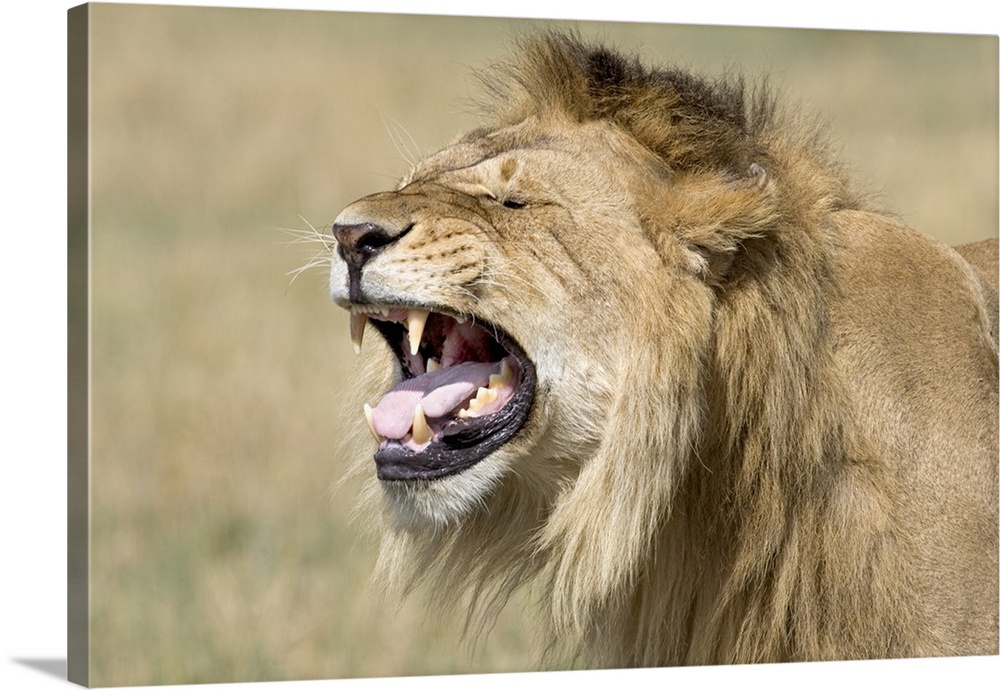This captivating piece of wall art, possibly printed on canvas, features a close-up, profile shot of a male lion centered in the image, facing the left. The lion appears to be either roaring or yawning, with his mouth wide open, revealing his sharp canine teeth and purplish tongue. His eyes are squinted shut, enhancing the intense expression on his face. The lion's mane is remarkably bushy and healthy, predominantly brown with hints of white, adding to his majestic appearance. Only the lion's face and the top of his body are visible, adorned with pronounced whiskers. The background is a blurred, brown-ish grassy area, suggestive of his natural savannah habitat, emphasizing the wild essence of the scene while maintaining a focus on the lion's powerful visage.